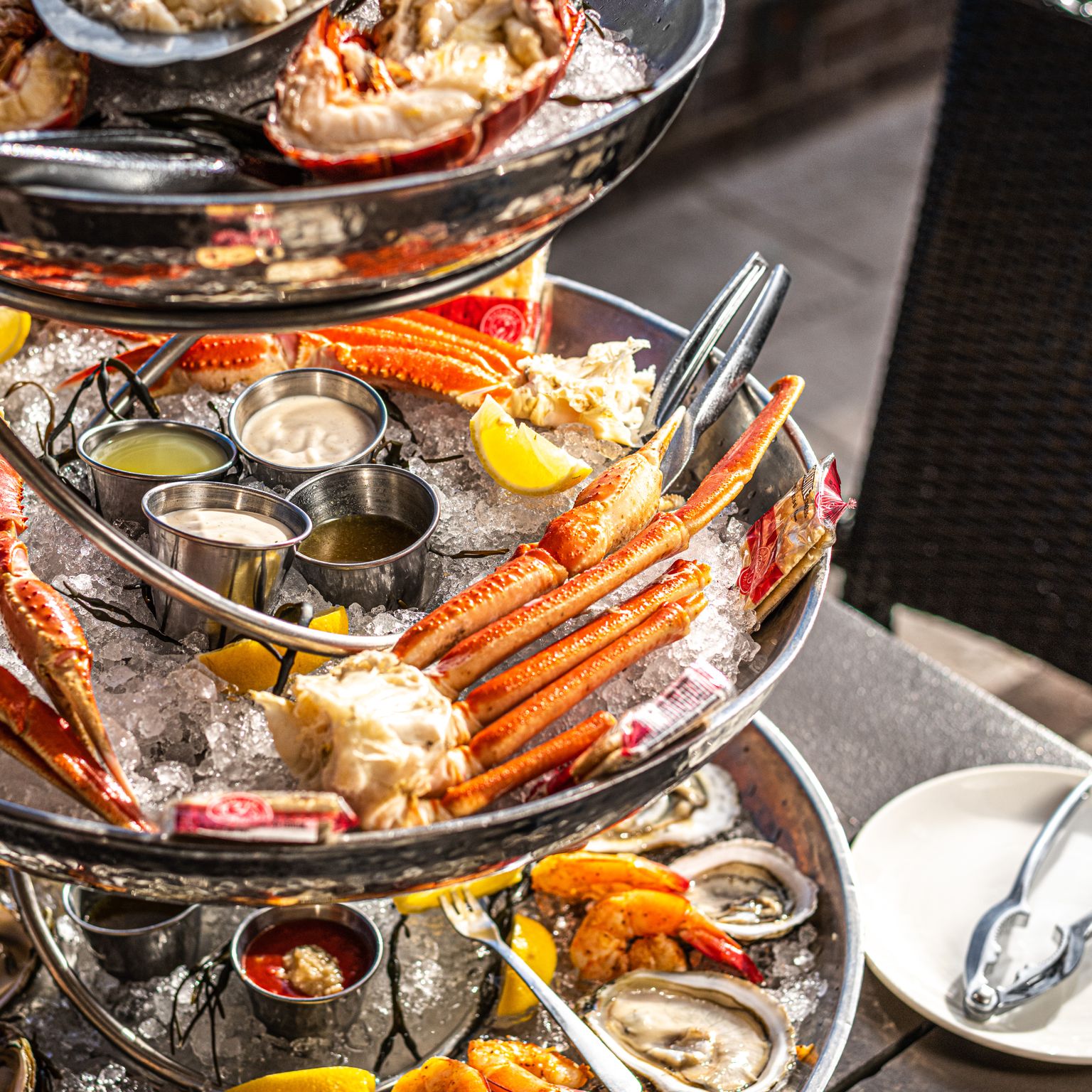This photograph captures an elegantly presented three-tiered silver serving tray filled with an assortment of fresh seafood kept crisp on beds of ice. The bottom tier features oysters on the half shell, whole and peel-and-eat shrimp, accompanied by lemon wedges and various dipping sauces, including cocktail sauce with horseradish and possibly butter. A small silver serving spoon is elegantly tucked into a lemon. The second tier showcases a generous portion of crab legs, also surrounded by ice and accompanied by four metal cups containing diverse sauces—likely butter, tartar sauce, and others that appear clear and white. The top tier, slightly cropped from full view, displays a succulent lobster tail, with a silver nutcracker placed nearby to crack open the shell. The entire stand rests on a beige table, and a dark brown rattan chair is partially visible in the background. To the right of the serving tray is a small white plate with another silver nutcracker tool, adding to the overall elegant seafood dining experience.